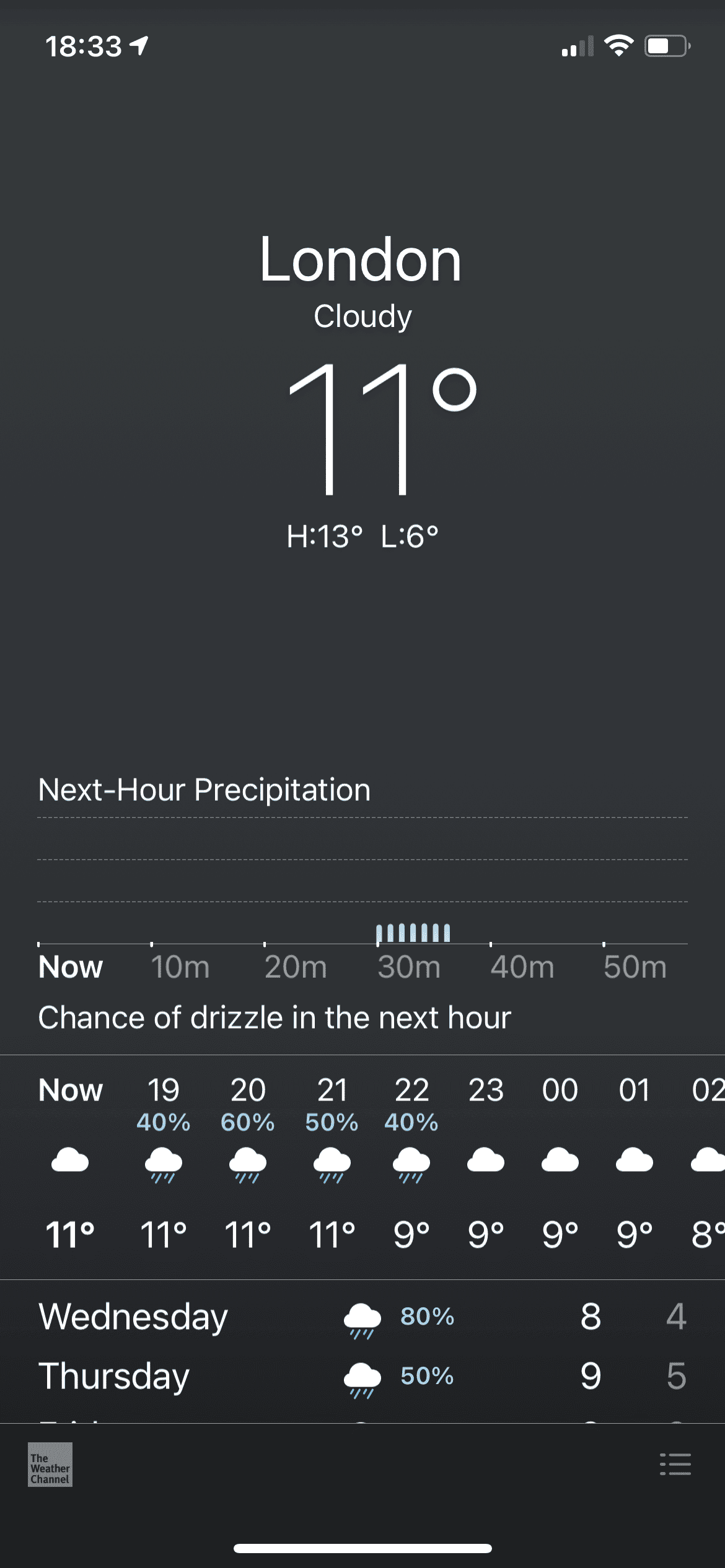This image is a vertically-oriented screenshot taken from a cell phone, displaying the weather application. The background is black with white text. In the top-left corner, the time reads 18:33, accompanied by a north-east facing arrow. The phone’s signal strength is shown with two bars, and the Wi-Fi symbol is visible. The battery indicator is half full.

Centered at the top, the location is listed as London, with the current weather described as cloudy, and a temperature of 11°C. The forecasted high is 13°C, and the low is 6°C. 

Midway down the screenshot, the "Next Hour Precipitation" section outlines the upcoming weather conditions by the hour. At 18:00, it is cloudy with a temperature of 11°C. By 19:00, there is a 40% chance of rain, signified by a cloud icon with raindrops, and the temperature remains at 11°C. At 20:00, the chance of rain increases to 60%, with the temperature steady at 11°C. The hourly forecast continues until 02:00, showing 8°C and cloudy conditions.

Beneath this, the forecast for Wednesday and Thursday is detailed. Wednesday has an 80% chance of rain with a high of 8°C and a low of 4°C. Thursday shows a 50% chance of rain with a high of 9°C and a low of 5°C.